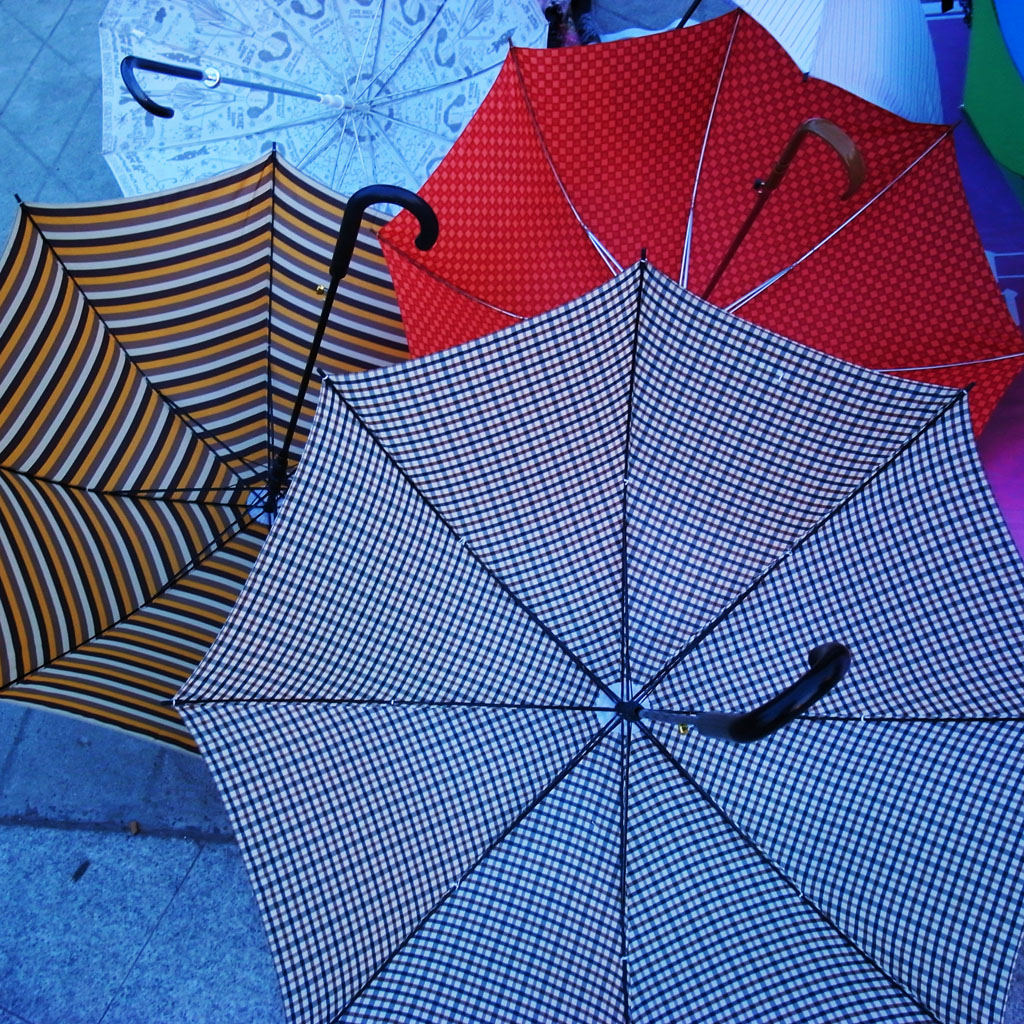In this photo, a variety of colorful umbrellas are arranged upside down on a tiled walkway, their black, curved handles pointing toward the sky. Dominating the scene, the vibrant umbrellas take up approximately 90% of the image, each displaying distinct and captivating patterns. In the upper left corner, a light blue umbrella stands out distinctly, while in the upper right, fragments of dark blue and green umbrellas are partially visible. On the left side, a striking umbrella with white, tan, and brown stripes draws attention, adjacent to another sporting a light and dark red checkered pattern. Close to the camera on the front right, a light blue and white checkered umbrella can be seen. Adding to the diversity, one umbrella features mustard, white, gray, and black stripes, while another bears a curious black and white line art depicting human-like figures. The scene is devoid of additional elements, focusing entirely on the umbrellas against a minimalist pale blue background.